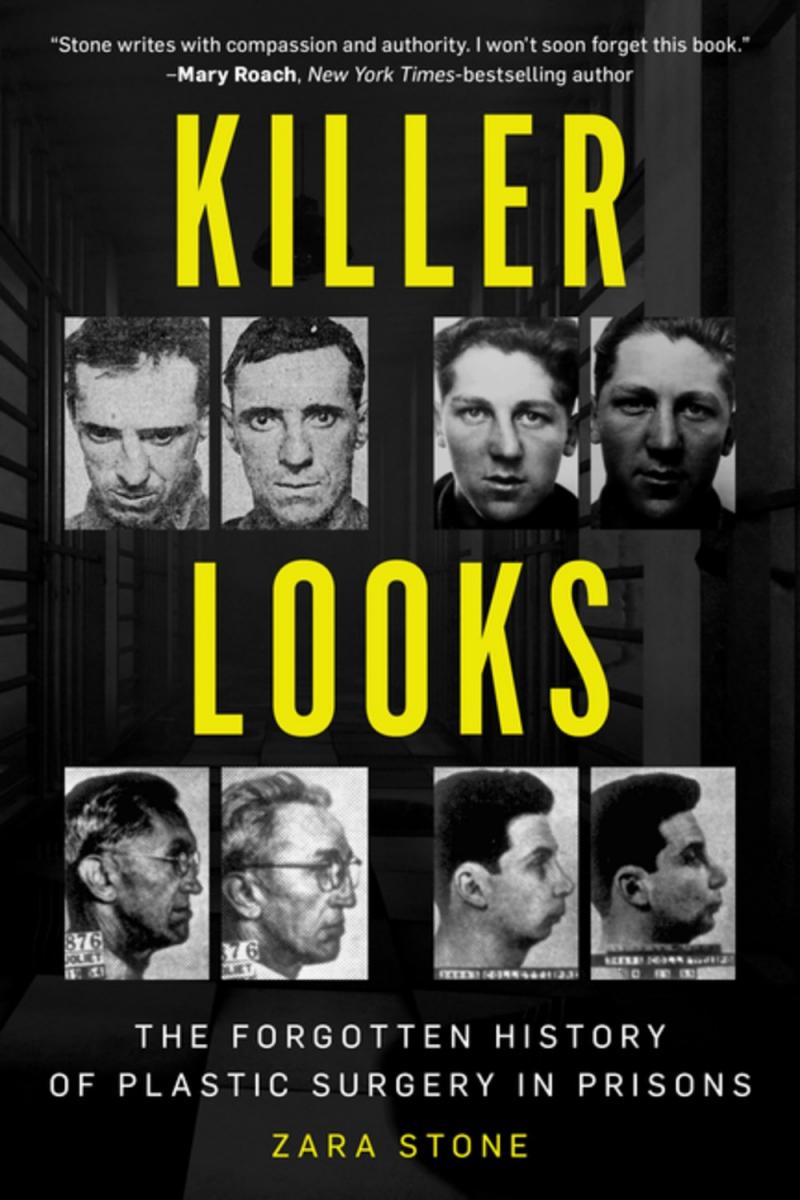The book cover is a compelling blend of vintage black and white photography and graphic design, set against a dark, faded background depicting a corridor of prison cells. Dominating the cover are two horizontal rows each containing four photographs, which are before and after images of four separate prisoners, showcasing noticeable changes such as a straightened nose. These black and white photos emphasize the thematic focus of the book.

Across the top in large, bright yellow, sans serif letters, the title "Killer Looks" draws immediate attention. Below the photographs, a white subtitle reads "The Forgotten History of Plastic Surgery in Prisons," conveying the book's intriguing subject matter. In smaller yellow text at the bottom, the author's name, Zarina Stone, is featured. Additionally, at the very top in small white text, a review by Mary Roach, a New York Times best-selling author, praises the book, noting, "Stone writes with compassion and authority. I won't soon forget this book." This meticulously designed cover effectively introduces the book's exploration of plastic surgery within the prison system.